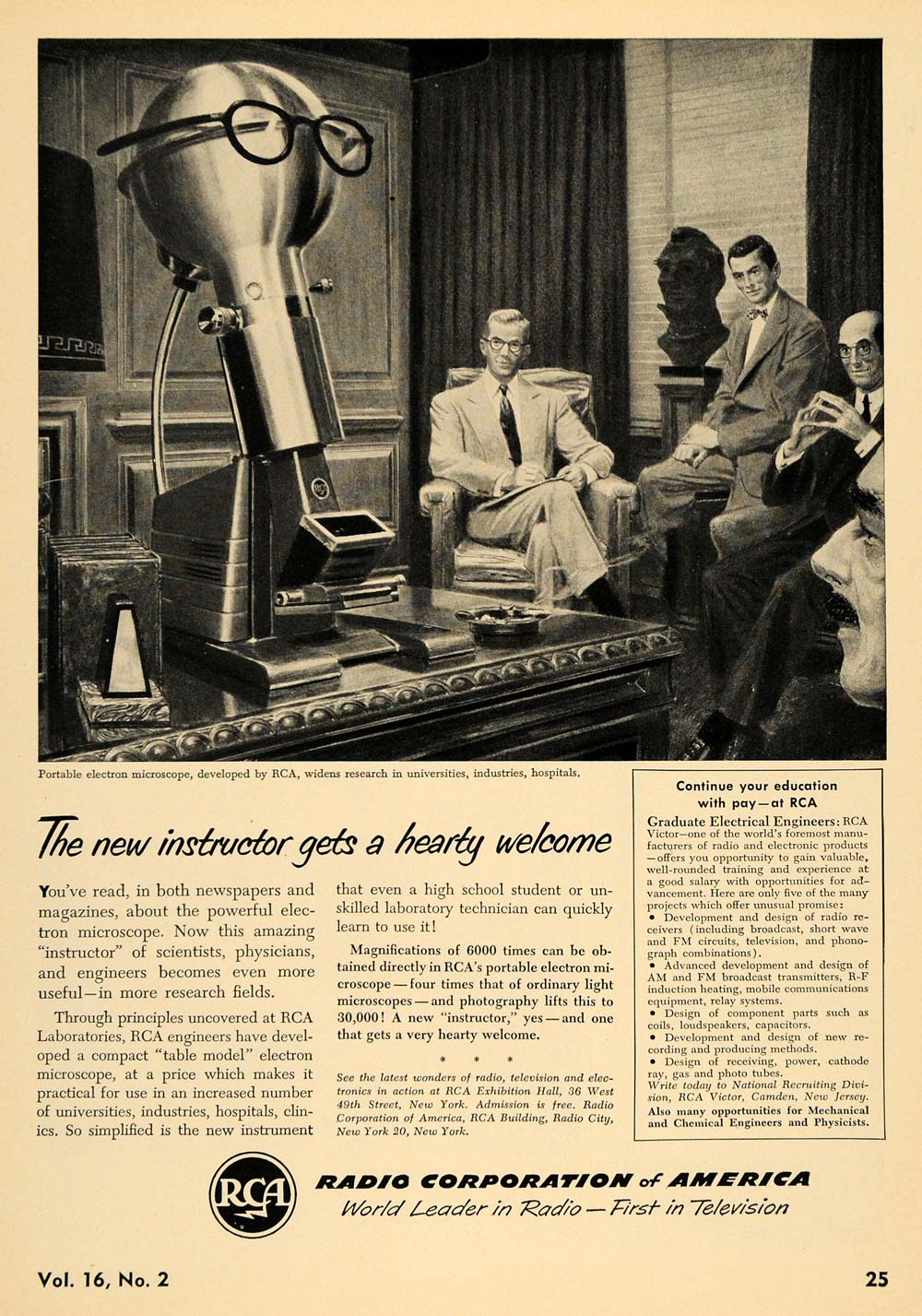The full-page advertisement, resembling an article from an old magazine circa the 1940s or 1950s, is printed on yellowed, beige-colored paper. Dominating the top half of the page is a detailed black-and-white illustration set against a wooden and curtained backdrop. In the illustration, a large robotic device with a spherical metal dome and black glasses, resembling a cross between a giant microphone and an industrial vacuum cleaner, sits atop a desk on the left side of the image. The desk also features an ashtray with a smoking cigarette. To the right, three men in suits and ties, with a fourth just visible on the extreme right, are seated and attentively observing the robot. Between two of the men, the bust of a statue can be seen. The headline beneath the illustration reads, "The new instructor gets a hearty welcome." Below, two columns of text explain the story, with a third column on the right bordered in black titled "Continue your education with pay at RCA." The bottom of the page features the RCA Victor logo, encircled with "Radio Corporation of America," and the tagline "world leader in radio – first in television." The lower left corner displays "Volume 16, Number 2," and the lower right corner is marked with the page number, 25.